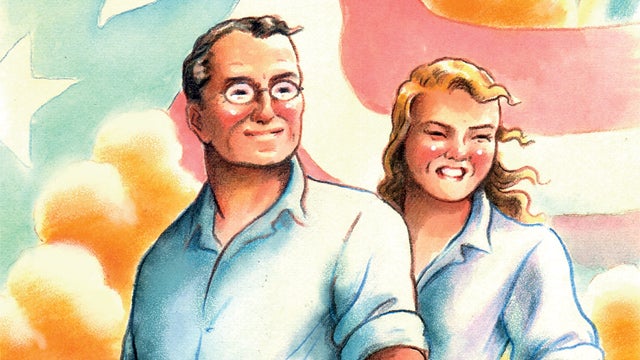This detailed illustration captures a man and woman standing together, depicted in a style that resembles early 1940s or 1950s artwork. Both characters are smiling and are of light skin complexion. The man, on the left, wears glasses, has short brown hair, and is dressed in a blue button-down shirt. The woman, on the right, has blonde hair flowing down her shoulders, rosy cheeks, and is also wearing a similar blue button-down shirt. Her mouth is open, showing her teeth, while the man's mouth is closed.

The background features a stylized American flag with light blue and red stripes, adorned with white stars on a blue field near the upper left of the image. Golden-yellow clouds also billow behind the characters, adding to the patriotic atmosphere. The entire scene is rendered in a colored pencil-like style, giving it a nostalgic, vintage feel. The two figures stand closely together, gazing towards the right side of the image, imparting a sense of unity and shared purpose.